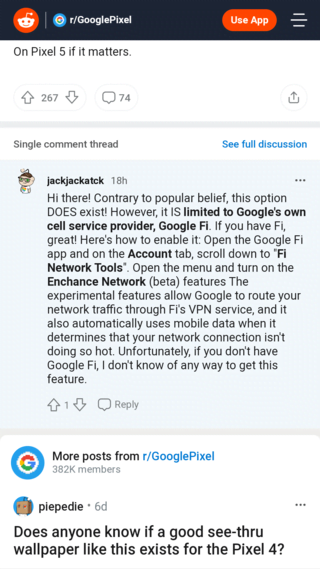**Caption:**
This is a detailed screenshot of a Reddit post discussing a feature specific to Google Pixel devices, particularly the Pixel 5. The post highlights a comment from a user named Jack, who clarifies that the option to enable certain networking features does exist but is exclusive to Google's cell service provider, Google Fi. Jack provides a step-by-step guide for Pixel users on Google Fi to enable the Enhanced Network beta: 

1. Open the Google Fi app.
2. Navigate to the Account tab.
3. Scroll down to Fi Network Tools.
4. Open the menu and activate the Enhanced Network beta.

The Enhanced Network beta allows Google to route network traffic through Fi's VPN service and switches to mobile data when the network connection is weak. Jack notes that this feature is not available to users who are not on Google Fi.

Beneath the main discussion, there is another post from r/GooglePixel featuring a user query about the availability of a see-through wallpaper for the Pixel 4, noted by a profile picture and timestamp from six days ago.